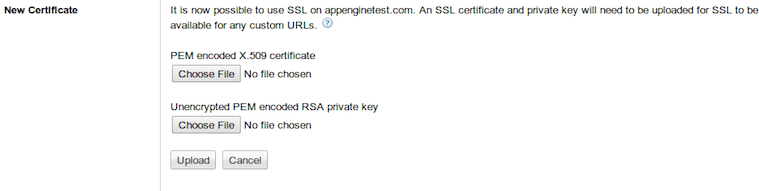This image, captured digitally, displays a user interface for uploading SSL certificates on the PenGenTest.com platform. In the upper left corner, there is a heading that reads "New Certificate" against a black backdrop. The screen is divided by a faint gray vertical line positioned slightly to the right.

The first section contains a message informing users that SSL can now be utilized on PenGenTest.com. It states, "An SSL certificate and private key will need to be uploaded for SSL to be available for any custom URLs." Adjacent to this message, a small question mark icon encircled is clickable, presumably for additional information.

Below this, a labeled space for uploading files is shown. It specifies "PEM ENCODED X.509 CERTIFICATE" in all capital letters. Next to a prompt that says "Choose File," the text "No file chosen" indicates that no file has been uploaded yet. Users can click on the "Choose File" button to select a certificate file from their device.

Further down, there is another upload section labeled "ENCRYPTED PEM ENCODED RSA PRIVATE KEY." This section also features a "Choose File" prompt and the corresponding indication "No file chosen."

At the bottom of the interface, there are two buttons: "Upload" and "Cancel," allowing users to either submit the selected files or abort the operation.